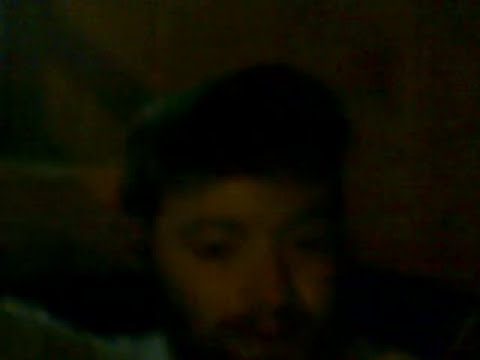The image is an extremely blurry photograph, potentially mistaken for a painting, featuring the close-up face of a man. His chin is cut off, and his overall appearance is very indistinct due to the blurriness. The man has a light complexion; although there is ambiguity regarding his exact ethnicity, he could be a light-skinned African-American or Hispanic. He seems to be wearing a black hat or possibly has very tall, puffy, or beret-like hair, high at the front and top and lower on the sides. He appears to have a beard and is not looking directly at the camera, but rather downward. The background is brown, resembling a wooden barn or an indoor setting, but remains indeterminate due to the darkness and lack of clarity in the image.